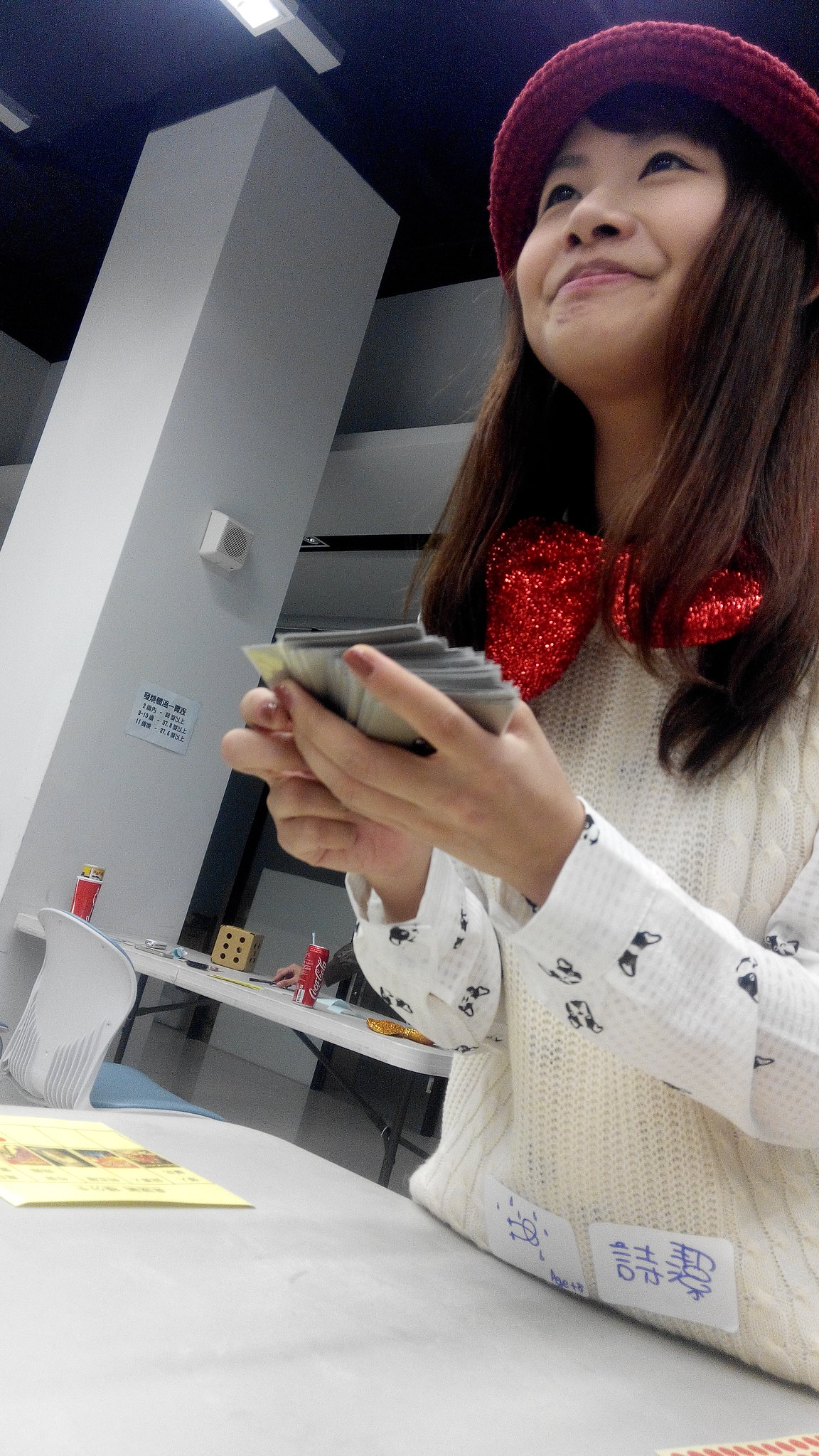At a bustling collectible card convention, a woman stands behind a plain gray fold-out table. Her attire is striking: she's dressed in a white long-sleeve shirt accentuated by an ornamental red bow tie and a maroon red beanie. Adding flair to her outfit, she wears an outer vest adorned with stickers featuring Asian characters. In her hands, she clutches a stack of collectible cards, possibly Pokemon or sports cards, attentively engaging with someone across the table.

The setting is modest, with another fold-out table visible behind her, accompanied by a simple chair and a blue cushioned seat. A familiar sight at such events, a Coke can and a Coca-Cola paper cup rest on the nearby table, hinting at the long hours spent at the convention. The detailed tableau suggests a vibrant, community-focused event where enthusiasts gather to share their passion for collectibles.